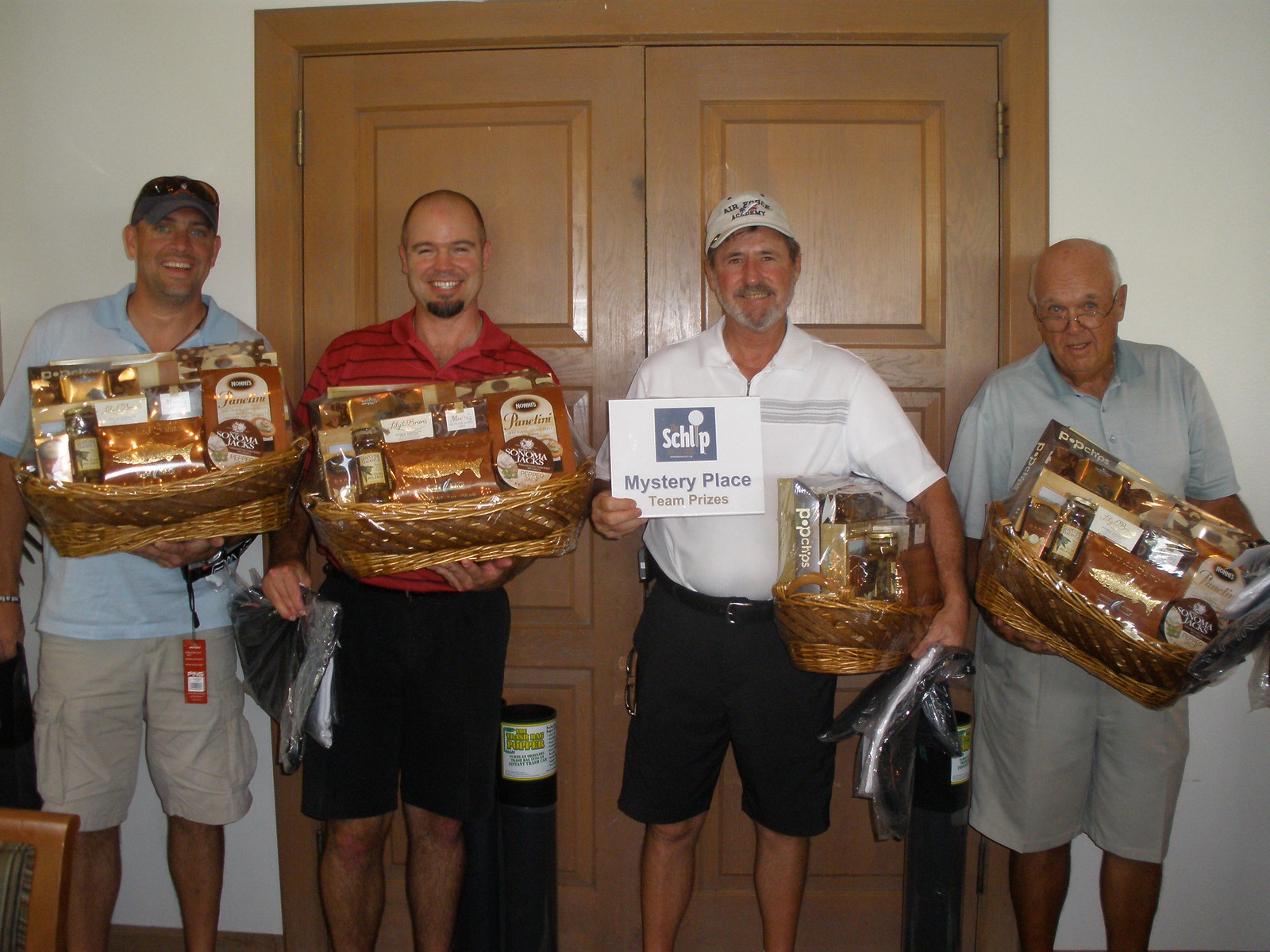This detailed photograph depicts four casually dressed men standing side by side in front of a wooden sliding doorway set into a white wall. They are all smiling and holding baskets brimming with assorted goodies like packets and small jars wrapped in plastic. The men are dressed in shorts and short sleeve shirts, exuding a relaxed and happy demeanor. Two of the men are wearing baseball caps, while the other two are balding, and none are wearing formal attire. The man in the center, dressed in a white short sleeve shirt and shorts, prominently holds a small sign that reads, "Mystery Place, Team Prizes." This unified group appears to be celebrating with their gift baskets, which seem to contain baked goods among other treats.